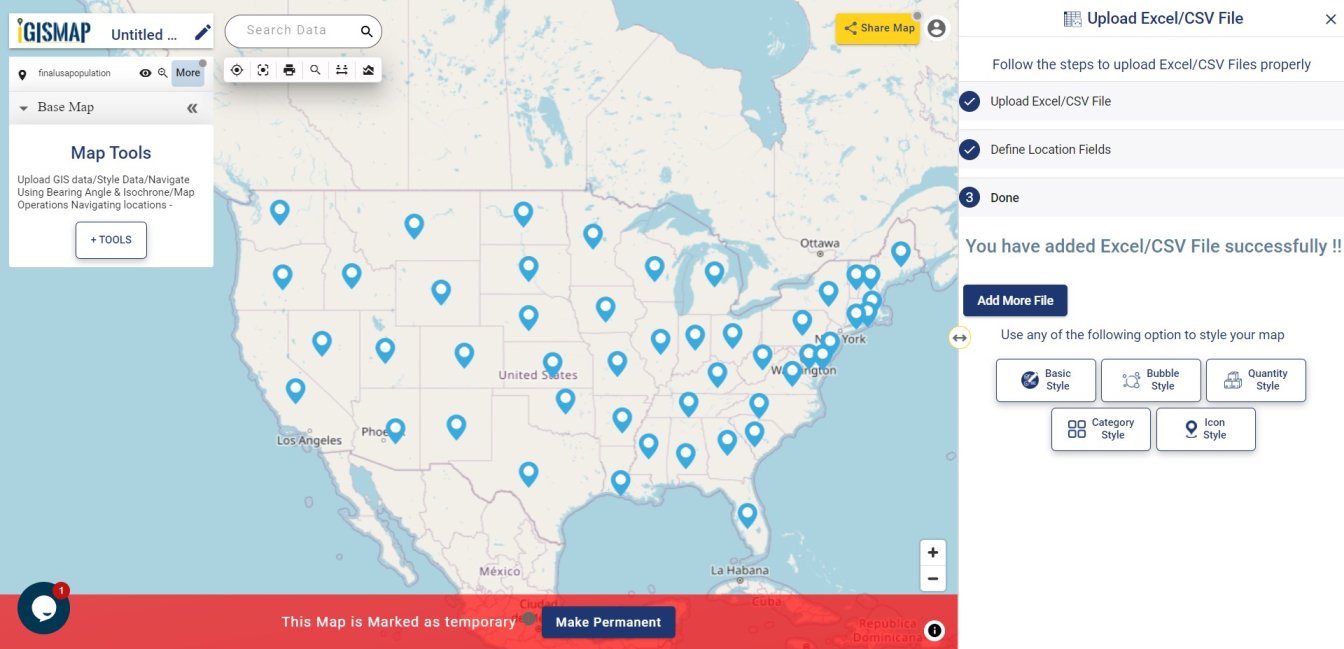On the left-hand side of the image is a continental map depicting the United States and Canada. Each continental state within the United States is marked with a blue GPS coordinate, though these coordinates are not necessarily positioned at the center of each state. In the upper left corner, there is a white section with green text that reads "GIS Map" and "Unedited." Additionally, there is some smaller, unreadable text beneath this heading.

Further down, there is a red background with white text in the center indicating, "This map is marked as temporary." Next to this, a blue button with white text reads, "Make Permanent." 

On the right-hand side of the image, instructions for uploading files are displayed. It states, "Upload Excel/CSV file. Follow the steps to upload Excel/CSV file properly." Below this, there are two blue check marks: the first one denotes "Upload File" and the second one instructs to "Define Location Fields." A third point, marked by the number three, says "Done." 

There is also an area designated for adding more files. Some blue rectangles with white interiors and blue text are presented here, though the text is unreadable due to the image size.

Transitioning from this section concludes the description of the image.